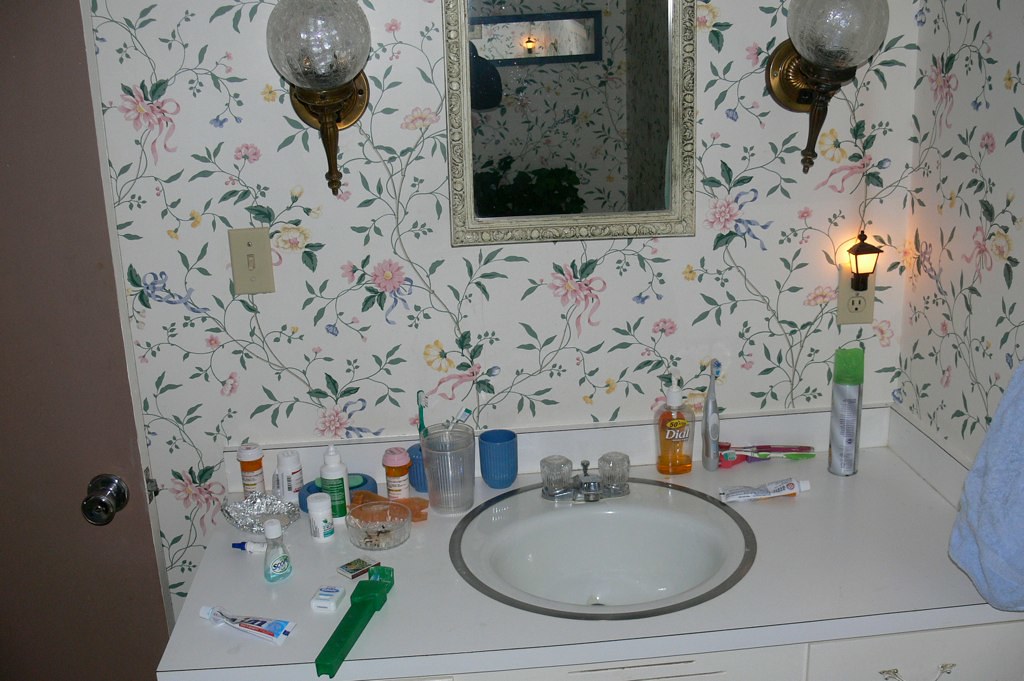This photograph captures an intimate glimpse into a small, vintage-style bathroom. Dominating the scene is a circular white ceramic sink, which features a silver outline and evokes a sense of nostalgia with its dated faucet. The faucet, harking back to designs from the 70s or 80s, boasts plastic, diamond-shaped turn knobs and includes a pull-up stopper for plugging the sink. 

The sink is set within a white, plastic laminate countertop, which holds a variety of everyday items scattered across its surface. Among the clutter are several pill bottles, a miniature bottle of Scope mouthwash with a small amount of green liquid remaining, and a green, square-shaped plastic toothbrush holder. An electric toothbrush stands near a nearly empty Dial soap dispenser, which contains a small quantity of orange soap at the bottom.

The backdrop of this bathroom scene is a white wallpaper adorned with a vibrant floral pattern. Pink daisies dominate the design, complemented by yellow flowers and intertwined with lush green vines, adding a touch of lively color to the room. This detailed and vivid description paints a comprehensive picture of the modest, yet nostalgically charming bathroom.